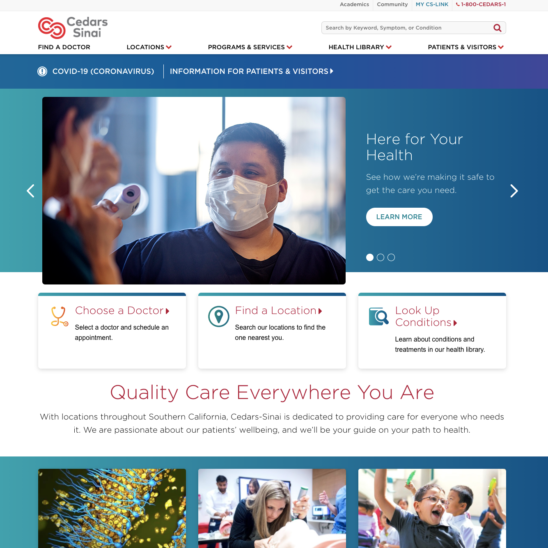The desktop version of the Cedars-Sinai website features a prominent display of the Cedars-Sinai logo, which resembles an infinity symbol composed of two red, curving lines forming an "S." The home page is designed with multiple sections, including options to find a doctor, locate medical facilities, explore programming services, access the health library, and navigate patient and visitor information.

At the center of the page, a stock photo showcases a patient wearing a white mask, accompanied by a message, "Here for your health. See how we're making it safe to get the care you need," along with corresponding call-to-action buttons such as "Choose a doctor" and "Find a location." Further down, a selection of additional stock photos with partially visible text underscores the institution's commitment to "Quality care everywhere you are," highlighting their extensive network across Southern California. Cedars-Sinai emphasizes their dedication to patient well-being and assures guidance on the path to health.

Additional website features include a convenient search bar located at the top-right corner and a contact number, 1-800-CEDARS-1, for easy access to support and inquiries.